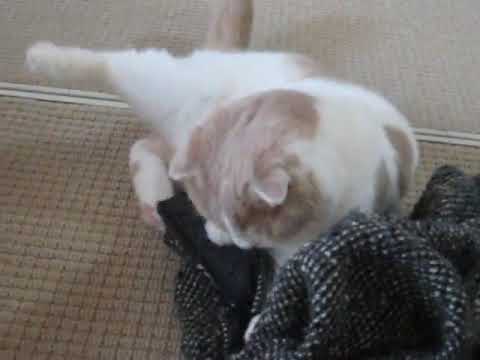In this image, we see a close-up of a mostly white cat with light brown patches on its head and back. The cat is positioned centrally, with its head slightly lowered, possibly looking down at something. The scene appears to be taken from above, revealing the cat sitting on a textured surface that has a grid pattern resembling an industrial fabric or carpet, with crisscrossed lines of a darker brown against a white and tan background. In the lower right-hand corner of the image, there is a gray, knitted garment, perhaps part of a person's coat or clothing, but without a clear presence of the individual. The colors in the image predominantly feature white, light brown, and gray, while the texture of the floor and the cloth contribute to a rich, detailed composition.